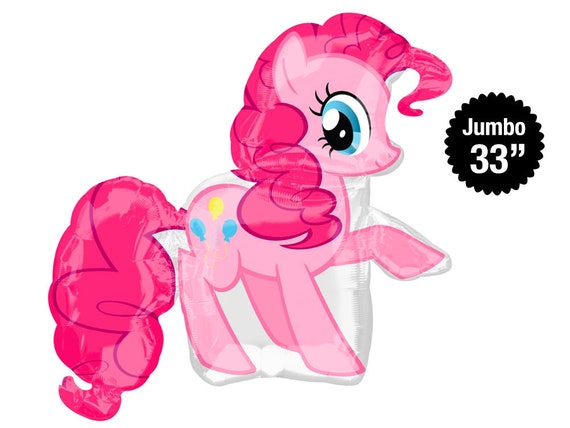This is a photograph of a jumbo 33-inch Mylar balloon featuring Pinkie Pie from My Little Pony. The balloon presents a profile view of Pinkie Pie, facing the right side of the image. The pony’s light pink body contrasts with its dark pink, fuchsia mane which, like her unfurled tail, has a shiny, slightly wrinkled appearance, typical of Mylar balloons. Pinkie Pie’s large, dewy blue eyes are detailed with three distinct eyelashes on both the top and bottom left sides. Her signature cutie mark, consisting of three balloons—two blue and one yellow—decorates her hip area. A black zigzag-edged starburst at the top right of the image announces the balloon’s jumbo size in white letters. The balloon’s ridged and glossy surface confirms its inflatable nature, and a hard edge runs along the pony's outline, hinting at the structural limitations of its design. Pinkie Pie's playful character is captured mid-step, with her front left hoof raised, while the other three hooves rest on the ground.